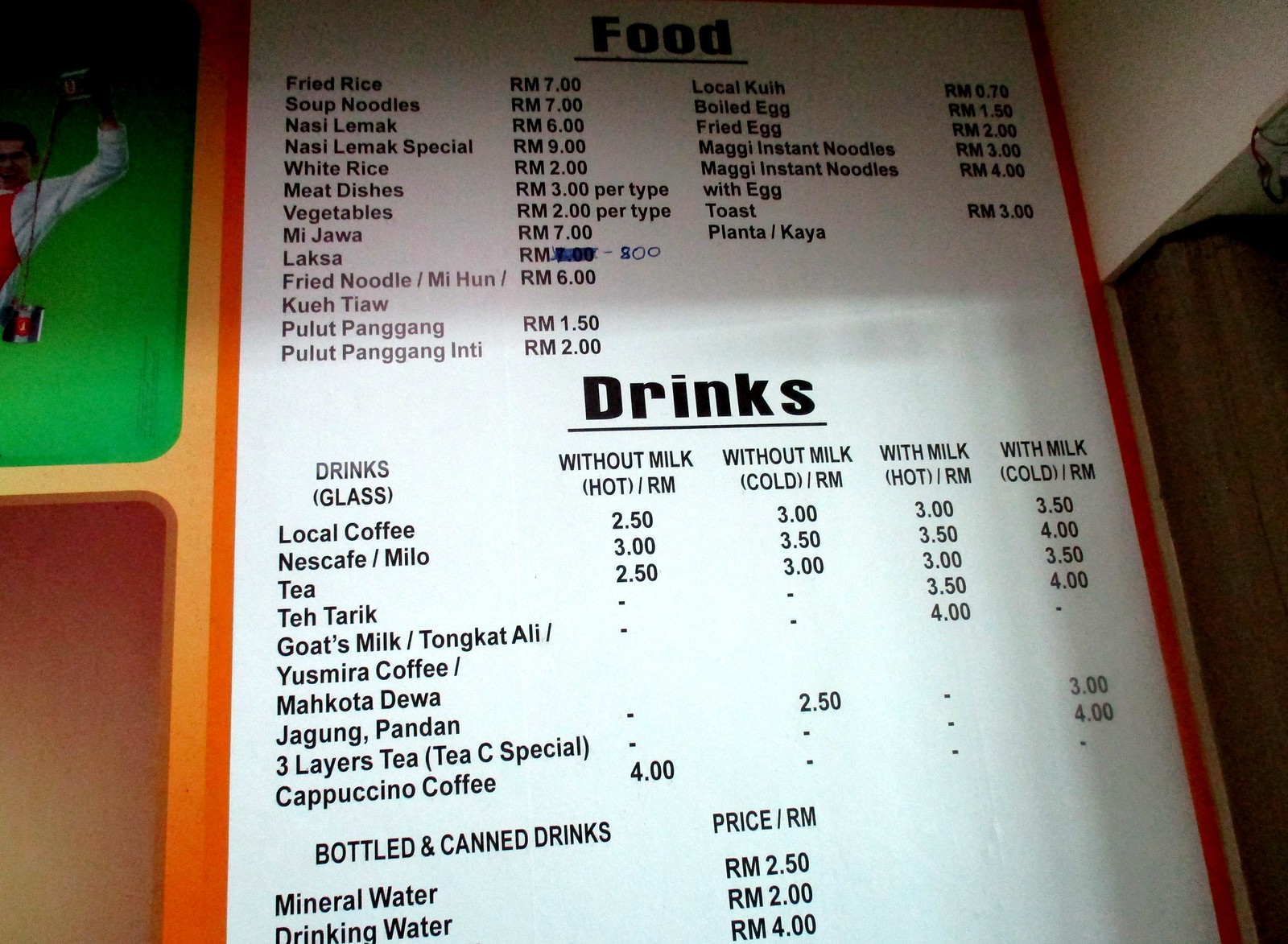This image captures a detailed menu mounted on a wall, characteristic of a Filipino or possibly an Asian restaurant, given the array of dishes and beverage options. The rectangular menu board, which is cut off at both the top and bottom, features a white background with bold black text. The top section of the menu prominently displays the title "Food," underlined in bold black letters. This section lists various dishes such as fried rice, fried noodles, pulut, and others, each with corresponding prices marked in the RM currency. 

Adjacent to the menu on the left is an orange-bordered sign, partially visible, featuring a green and a brown image. To the right, part of a white corner is layered over a brown wooden surface. 

Below the food section, there is another large underlined title, "Drinks," beneath which the menu is divided into multiple columns detailing different beverage options. These include local coffee, tea, usmira coffee, and makota diwai, each listed with variations like without milk hot, without milk cold, with milk hot, and with milk cold, along with their respective prices. Further down, a distinct "Bottled and Canned Drinks" section lists items such as mineral water and drinking water.

Additionally, noticeable details include small complex images within the menu and a partially visible green picture of a man in the upper left corner, possibly holding a fishing rod. This highly detailed depiction suggests the menu offers a broad selection of food and drink, catering to various preferences.